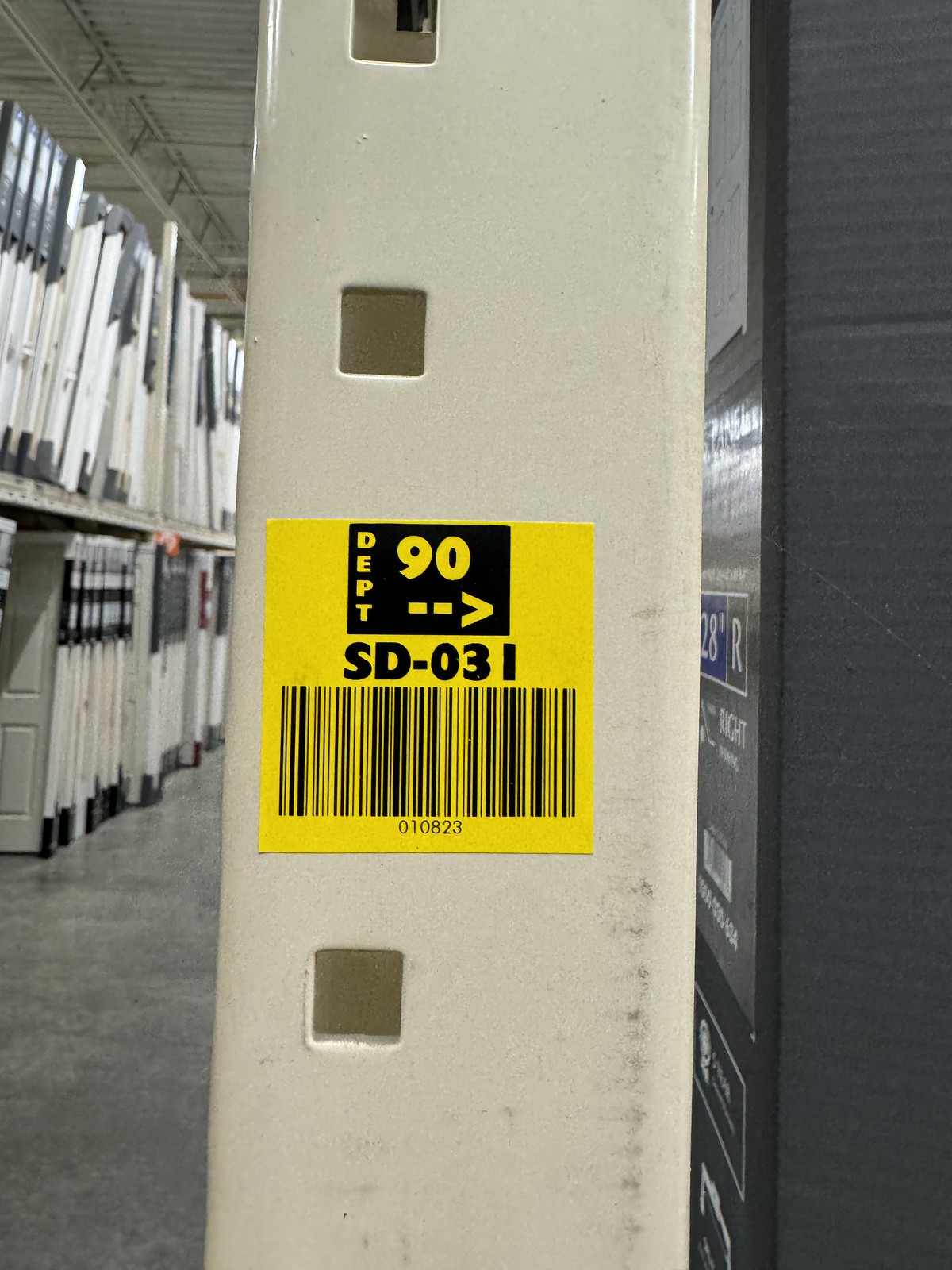The photograph captures an interior scene from within a store, predominantly showcasing a shelving unit. The background is lined with additional display shelves, which feature what appear to be multiple doors, stacked upright in a manner similar to books on a shelf. 

The focal point of the image is a vertically-oriented leg of one of the shelving units, rendered in a tan-grayish hue and prominently occupying most of the frame from top to bottom. On the left side of this shelving leg are three square holes arranged vertically. The top two holes are positioned closely together, while a third hole is situated further down, separated by a visible gap. 

Within this gap, the visibility of another potential hole is obstructed by a yellow sticker. This sticker contains several elements: a black barcode, a black square with yellow letters reading "90 departments," and an arrow pointing to the right. Below these elements, the sticker has the text "SD-031" in black. 

The image is somewhat perplexing due to the specificity of its subject matter—the shelving leg—but these details collectively form a curious and detailed glimpse into the scene.